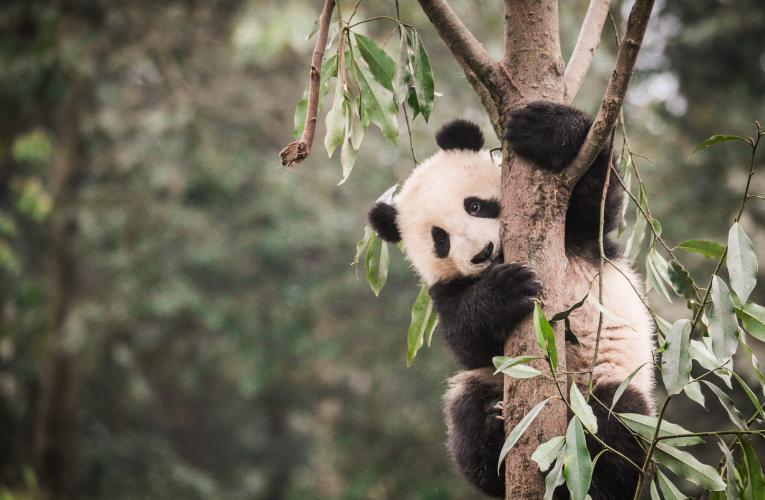In this vibrant color photograph, a playful panda cub is seen clinging to a slender tree trunk situated on the right side of the image. The cub's fluffy body is securely wrapped around the tree, with one arm confidently grasping a branch above, resembling an outstretched arm, while the other arm encircles the main trunk. The panda's small eyes, ears, arms, and legs exhibit their characteristic black coloration, contrasting vividly with its white face and belly. The young panda gazes curiously into the camera, creating an endearing focal point. Surrounding the subject, the out-of-focus background reveals additional trees with lush, green, narrow, and pointed leaves, adding depth and a sense of natural habitat to the composition. The tree's bark is a rich brown, providing a warm, earthy contrast to the panda's monochromatic fur.